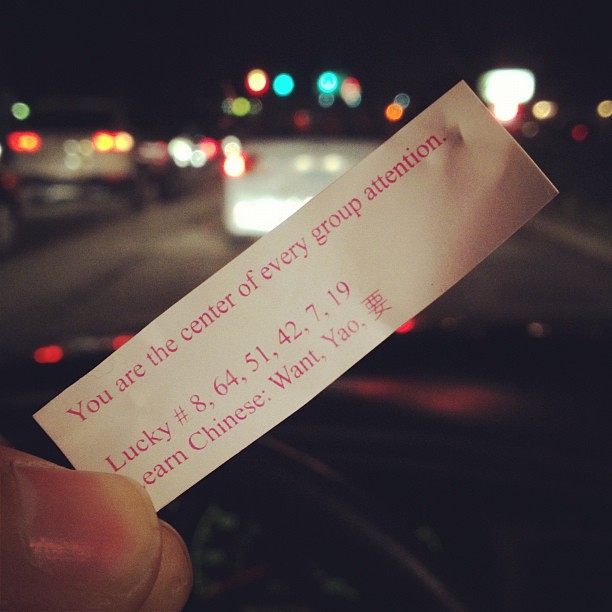This close-up image captures a small rectangular slip of paper from a fortune cookie, held between the left thumb and index finger of a white person. The fortune, printed in pink text on a white background, reads, "You are the center of every group attention." Below this, it lists lucky numbers—8, 64, 51, 42, 7, and 19—and includes a "Learn Chinese" section that teaches the word "want" (yao), along with the corresponding Chinese character. The photograph is taken inside a car at night, evident from the blurred background showing city lights, a gray truck, and heavy traffic. Reflections of the night sky and various vehicles' lights can be seen through the windshield, with a black steering wheel and dashboard visible in the foreground. The focus remains sharply on the fortune slip, with the car interior and outside scene softly out of focus.